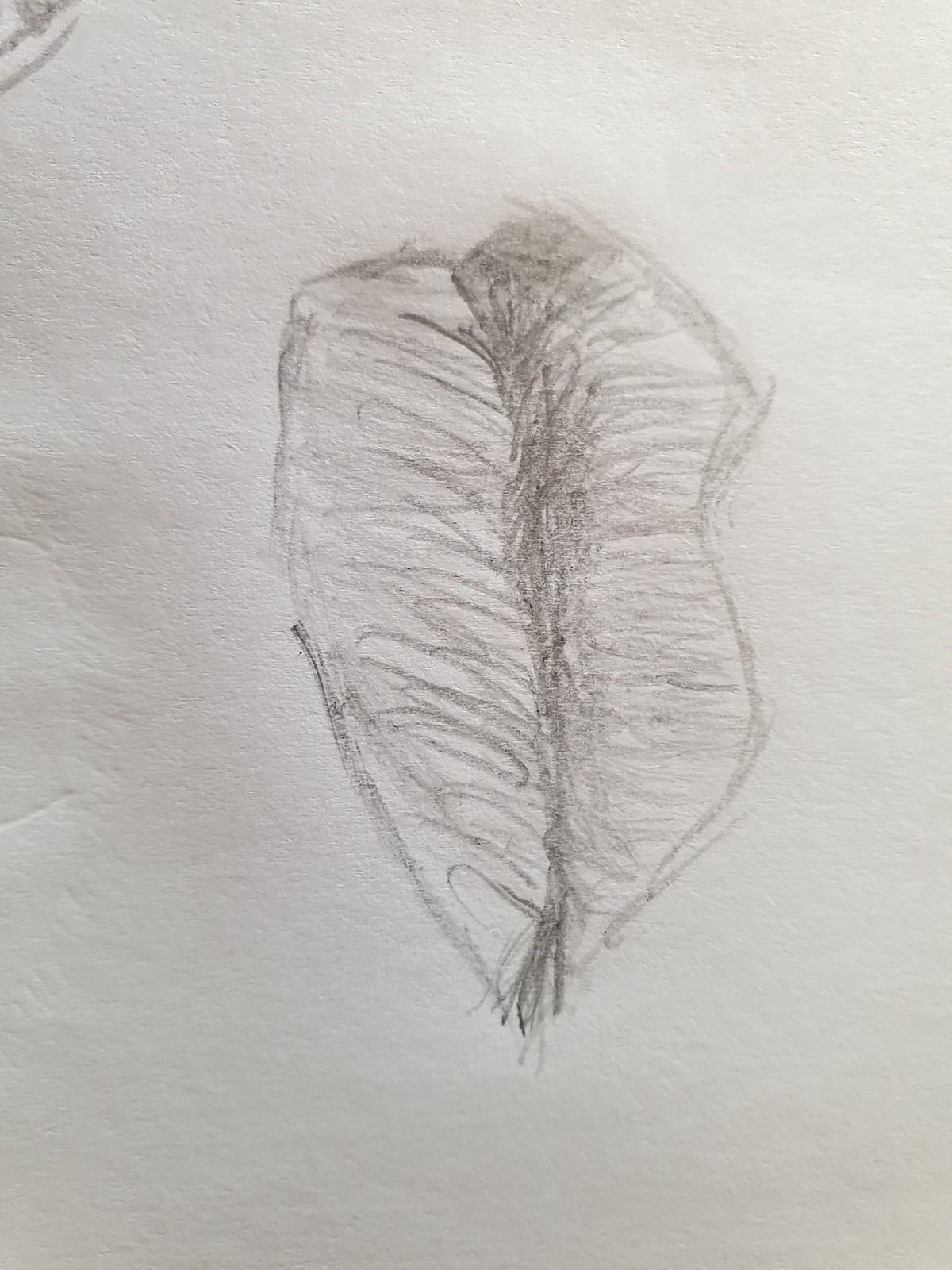A pencil sketch on a white sheet of paper depicts a rough, scribbled outline that most likely represents a pair of lips, although there is some confusion about its intended subject due to the crude execution. The sketch portrays the lips in a sideways orientation, with heavy shading between the lips and a noticeable M shape in the upper lip. The overall image is simplistic and lacks symmetry, leading to varied interpretations, such as a leaf or a scar. Some dark lines and shading fill the shape, with additional tiny pencil markings in the upper left corner of the paper. Despite its ambiguity, the drawing invites intrigue through its textured, scribbled details and heavy shading.